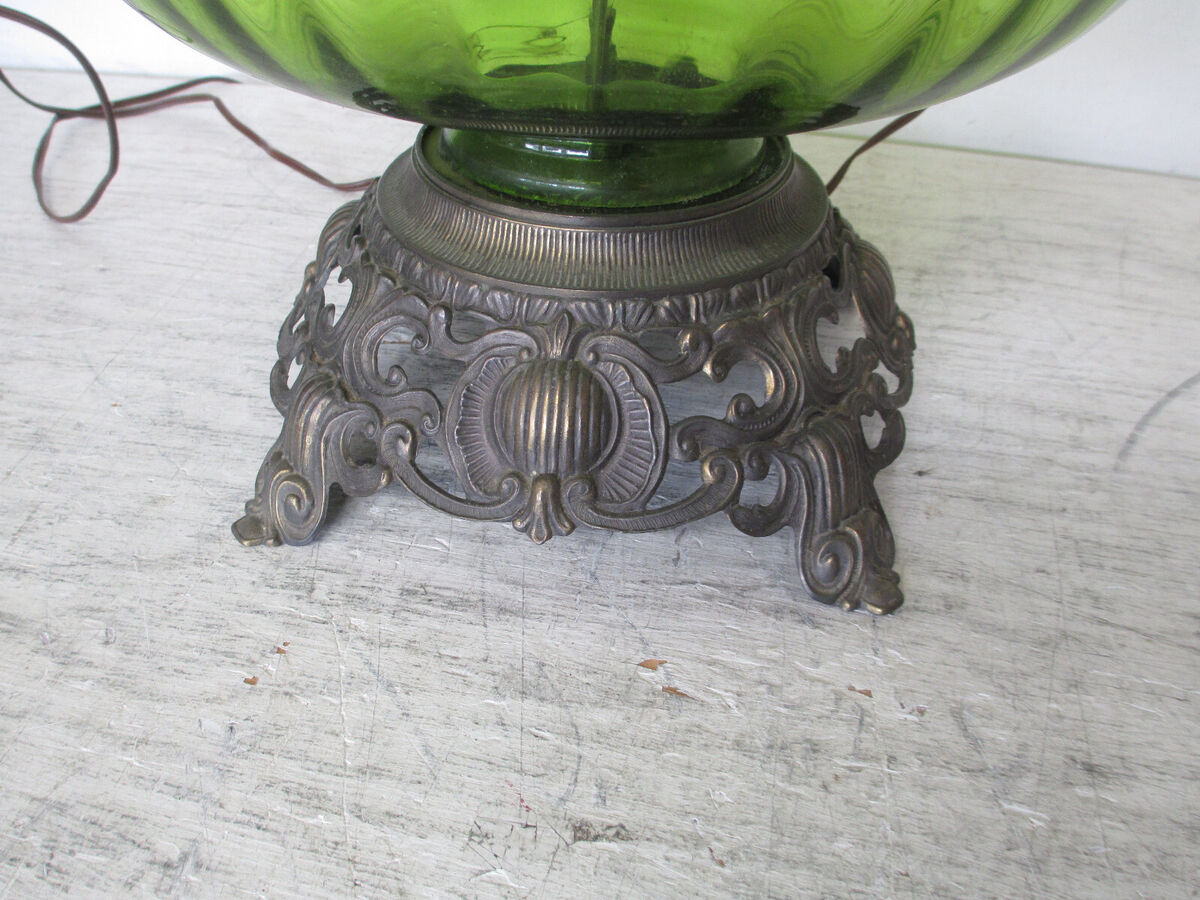In this close-up photograph, the scene is dominated by the ornate base of what appears to be an antique lamp. The base, resting on a distressed and chipped white-painted wooden table, is a tarnished bronze color, although it could be made of plastic with a metallic coating. The base itself is circular with intricate swirls resembling shells or waves and features four legs, of which only the front two are visible. A thin brown electrical cord extends from the back of the base, confirming its function as a lamp. At the top of the base, the bottom edge of a transparent green glass globe is visible, but the image is cut off above that point, leaving the full shape of the globe to the imagination. The background reveals a white wall, suggesting the table is positioned directly against it. The photograph captures the base and partial globe in great detail, emphasizing its aged and potentially antique aesthetic. The overall tilted composition of the image adds a dynamic touch to the scene.